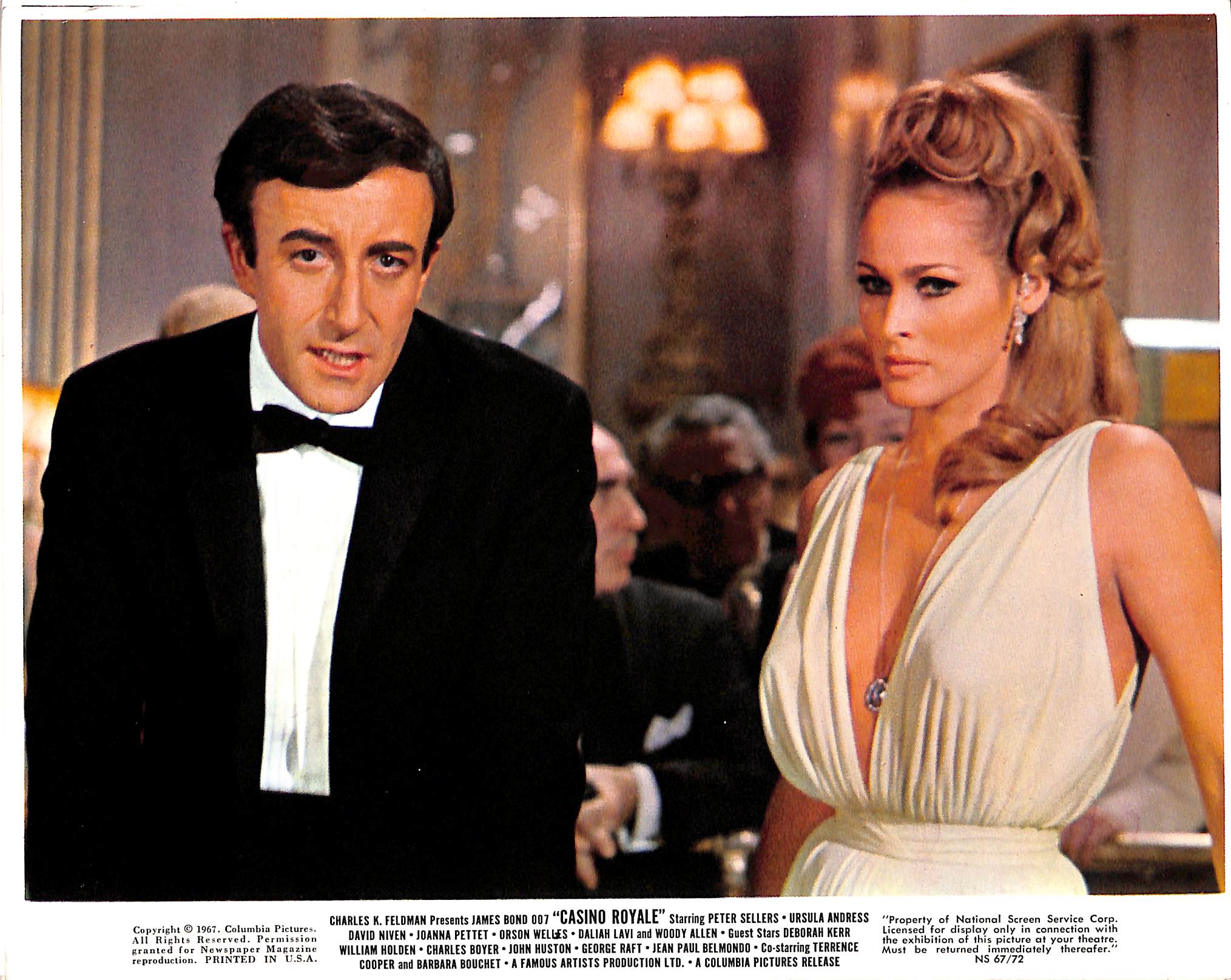This is a detailed color photograph and advertisement for the movie "Casino Royale," likely from the 1960s, featuring Columbia Pictures copyright information. The image highlights two prominently dressed figures. On the left is actor Peter Sellers, clad in a sophisticated black dinner jacket with a subtle pattern, a white button-up shirt, and a black bow tie. He sports a neat, short black hairdo. To his right stands an elegantly dressed woman with a glamorous updo cascading down her shoulder. She adorns a light ivory, sleeveless halter top dress with a plunging neckline, showcasing a silver necklace and diamond earrings. Her dress tightens around the waist and flows downward elegantly. Between them, an older gentleman looks off to the side, and in the background, people in formal attire are seen seated in a richly paneled room with illuminated wall sconces. Below the image, text prominently displays the movie title "Casino Royale" and features the names Peter Sellers, Ursula Andrus, David Niven, and Joanna Pettet in larger letters, hinting at a classic film ambiance.